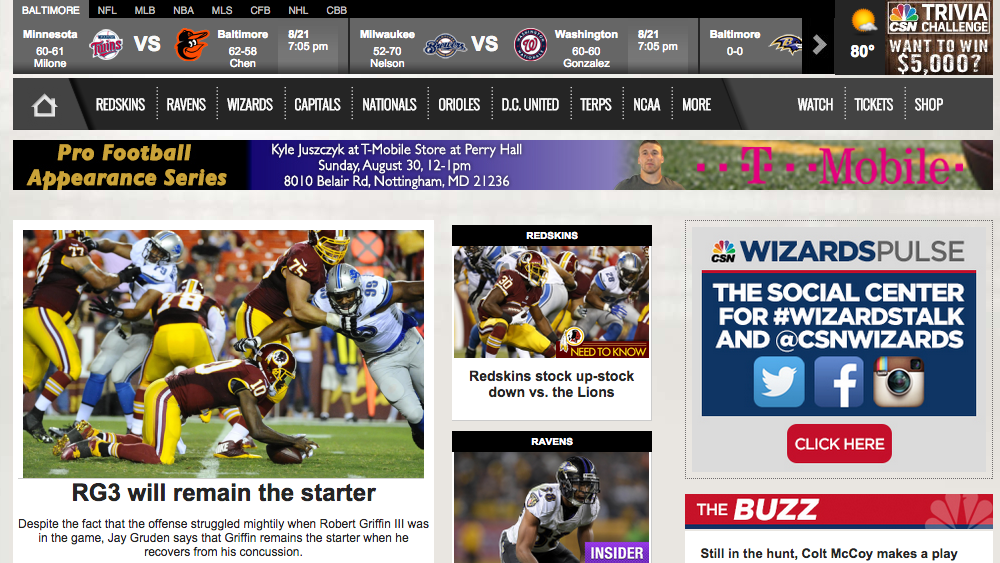**Descriptive Caption:**

The image is a screenshot taken from a news website on a laptop in landscape mode. In the upper-left corner, the page is labeled "Baltimore," flanked by tabs for various sports leagues: NFL, MLB, NBA, MLS, CFB, NHL, and CBB. The upper-right corner of the page features a weather update for a mostly sunny day at 80 degrees and a promotion for the "CSN Challenge" with a chance to win $5,000.

The top row displays an upcoming baseball game: Minnesota vs. the Baltimore Orioles, with team records listed as 60-61 for Minnesota and 62-58 for the Orioles, scheduled for 8/21 at 7:05 p.m. 

Below this, there's a navigation bar with tabs such as Home, Redskins, Ravens, Wizards, Capitals, Nationals, Orioles, DC United, Terps, NCAA, More, Watch, Ticket, and Shop.

In the second row, an announcement is made for a pro football appearance featuring Kyle Juszczyk of the Redskins at a T-Mobile store in Perry Hall on Sunday, August 30th from 12 to 1 p.m. The address is provided: 8010 Bel Air Road, Nottingham, Maryland, alongside a picture of Kyle at a T-Mobile store.

Further down, there are various sections of the page featuring different images. One section includes football images with headlines stating "RG3 will remain the starter" and "Redskins stock up, stock down vs. the Lions." Another section is dedicated to the "CSN Wizards Pulse," a social center for discussing the Wizards, with icons for Twitter, Facebook, and Instagram shown next to it.